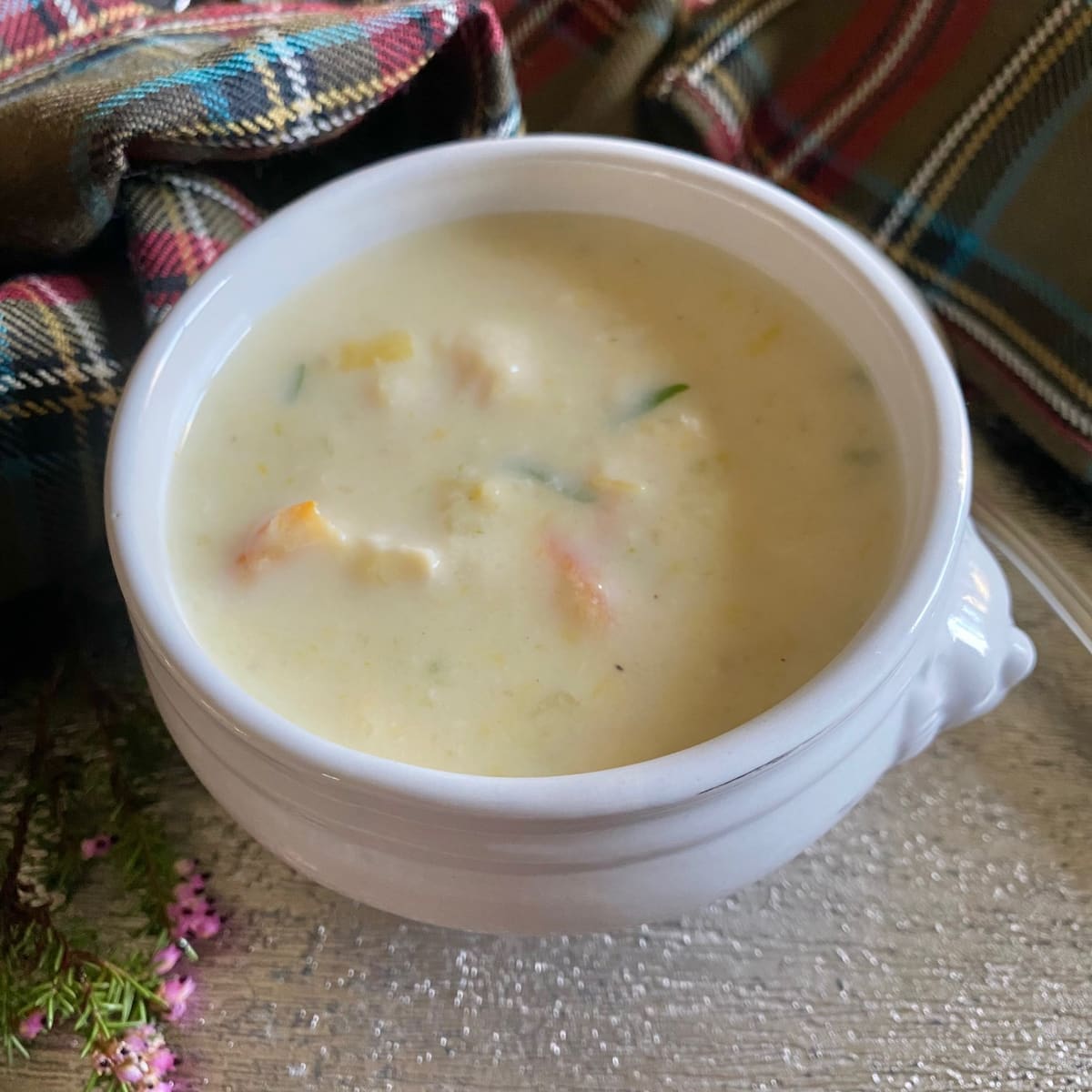This square color photograph features a detailed and visually appealing image of a delicious, creamy bowl of soup, possibly a corn or clam chowder. The light yellow soup is served in an ornate white ceramic bowl, which features a decorative protruding element resembling a flower. The soup contains visible pieces of orange-colored shellfish or carrots, green herbs or chives, and possibly potatoes, adding variation to its texture. The bowl is placed on a silver table, adorned with small pink and purple flowers thoughtfully arranged beside it. A multicolored tartan plaid blanket in shades of red, green, yellow, white, blue, and black provides a cozy backdrop, partially rolled and draped around the bowl, enhancing the warm, inviting appearance of the setting. The absence of steam suggests a photo captured at room temperature.